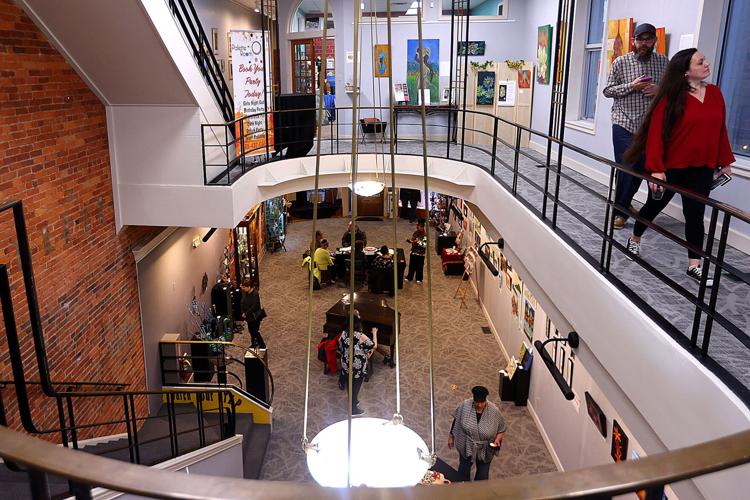A photograph captures a bustling art gallery or museum from an elevated vantage point atop the staircase, revealing both the first and second levels. The lower floor showcases an array of paintings adorning the walls, highlighted by strategic lighting, with people milling about, examining the artworks. Central to the scene is a grand piano and a registration desk where individuals are seated. Entry doors are visible, welcoming visitors in. Parallel staircases, separated by a red brick wall, connect the two levels. The second floor features more large paintings and a poster advertising an upcoming event. There's a gray-carpeted hallway with a railing, where a woman in a red shirt and a man with a checkered shirt and beard walk by. The atmosphere is lively, with approximately ten people dispersed throughout the space, immersed in the art around them.